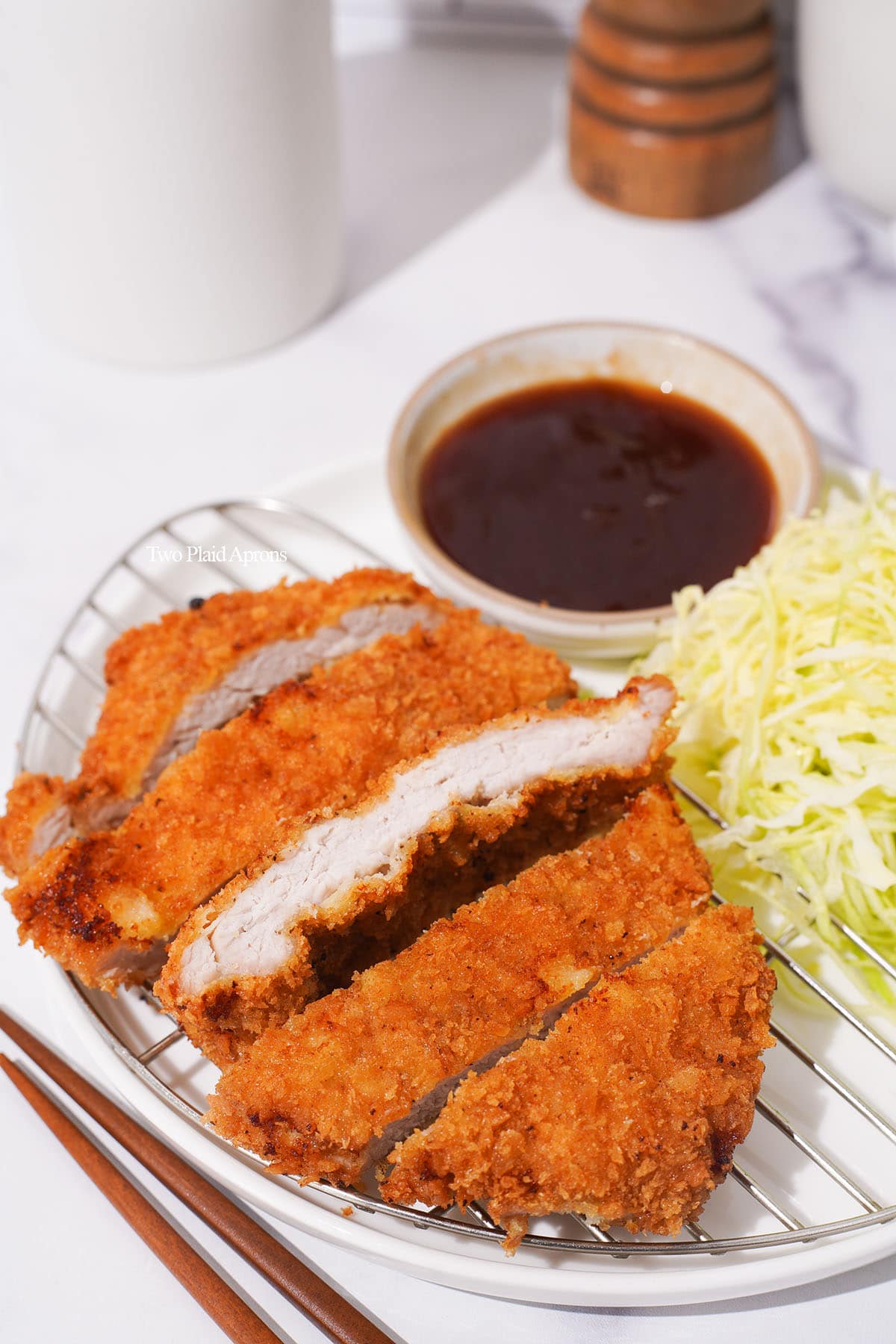The image depicts a zoomed-in view of a plated meal against a white tablecloth on a stone countertop with gray veins. At the center of the white plate lies a deboned, golden brown, crispy-coated chicken breast that has been sliced and placed on a half-moon-shaped metal cooling rack. To the side of the chicken is a serving of off-white noodles or possibly cabbage with a green tinge, resembling coleslaw. Adjacent to the noodles/cabbage, a small bowl contains a dark reddish-brown sauce with a textured appearance. A pair of brown chopsticks rests on the left side of the plate, hinting at an oriental-style meal. In the background, there are salt and pepper shakers and two jars, one ceramic and one wooden, completing the scene.